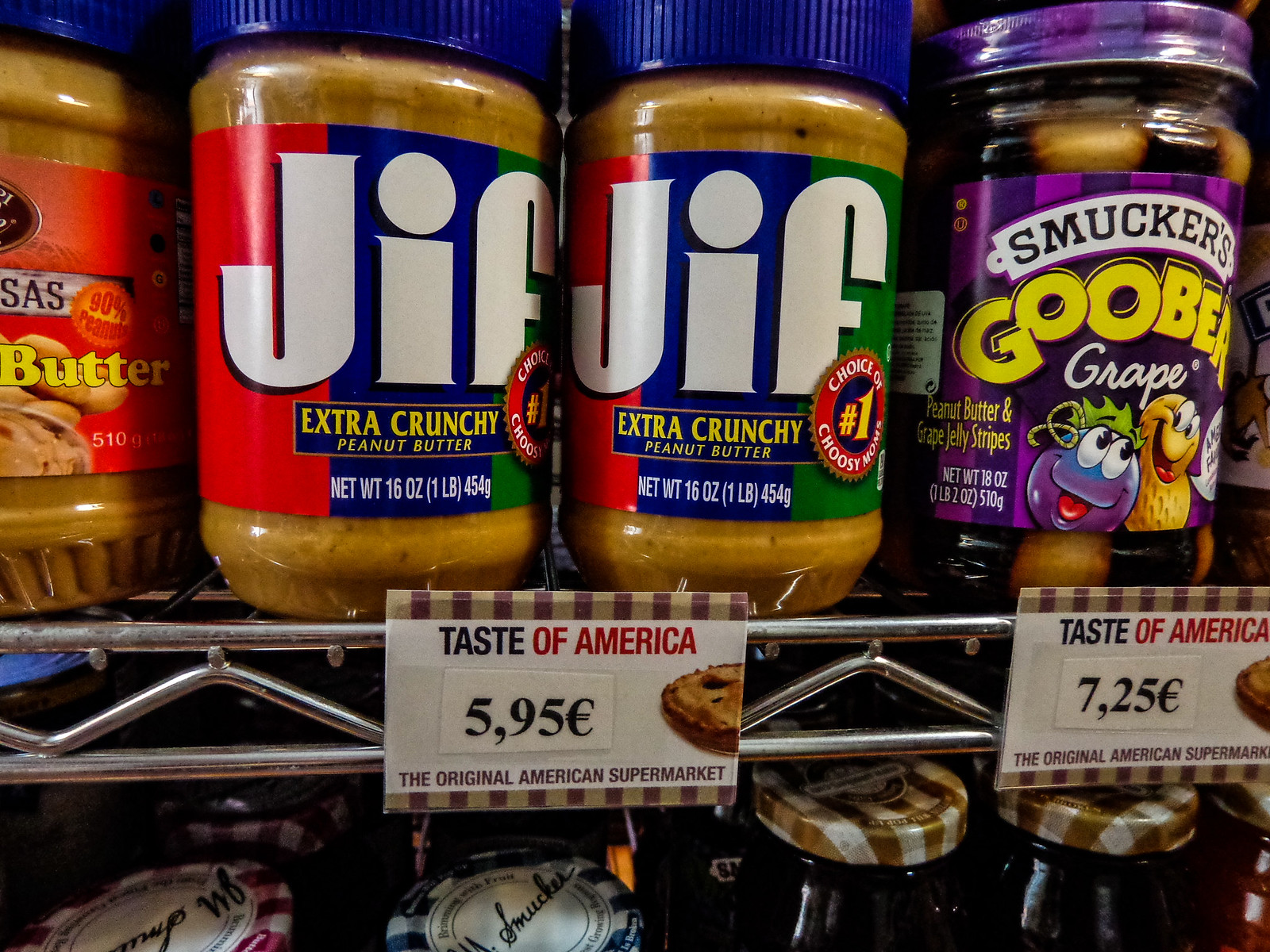The image shows a shelf in an international supermarket, featuring American products. There are two jars of Jif Extra Crunchy Peanut Butter on the left, each with blue lids and labeled as 16 ounces (1 pound). To the right, there's a jar of Smucker's Goober Grape, which combines peanut butter and jelly in one, with a distinctive purple lid. In front of these products, there's a label reading "Taste of America" in black and red letters with an image of an apple pie. The price for the Jif peanut butter is listed as €5.95, while the Smucker's Goober is priced at €7.25. The labels indicate that this section is part of the "Original American Supermarket" section, hinting that these products are imported and highlighted for their American origin. Additional jars of jelly can be seen at the bottom of the shelf, though only the tops are visible.